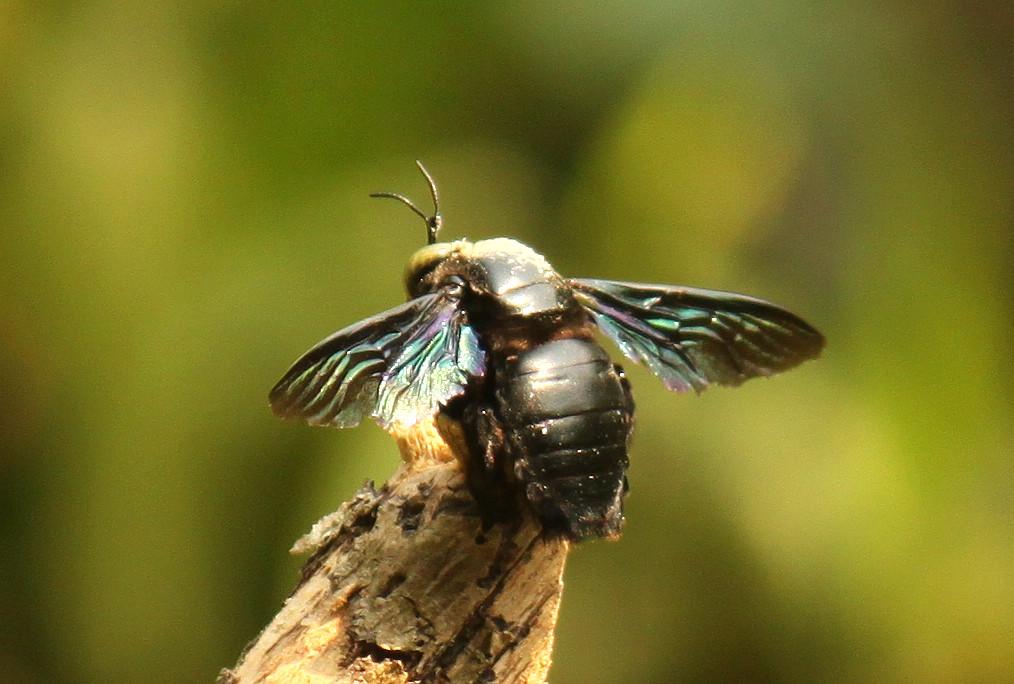In this close-up color photograph, we see a bee-like insect perched on a piece of flaky wood, facing away from the camera. The insect has an iridescent shine to its wings, displaying vibrant teal, purple, and yellow hues. Its body is predominantly shiny black, and the back section is notably large. The wings, though small in comparison to its body, include two larger and two smaller ones with a shimmery appearance that ranges from dark purple to green. Two black antennae protrude from its head, pointing forward. The wood it rests on features a mix of dark brown, lighter brown, and beige tones. The background is entirely out of focus, rendered in various shades of green, adding a soft, natural backdrop to the detailed foreground.